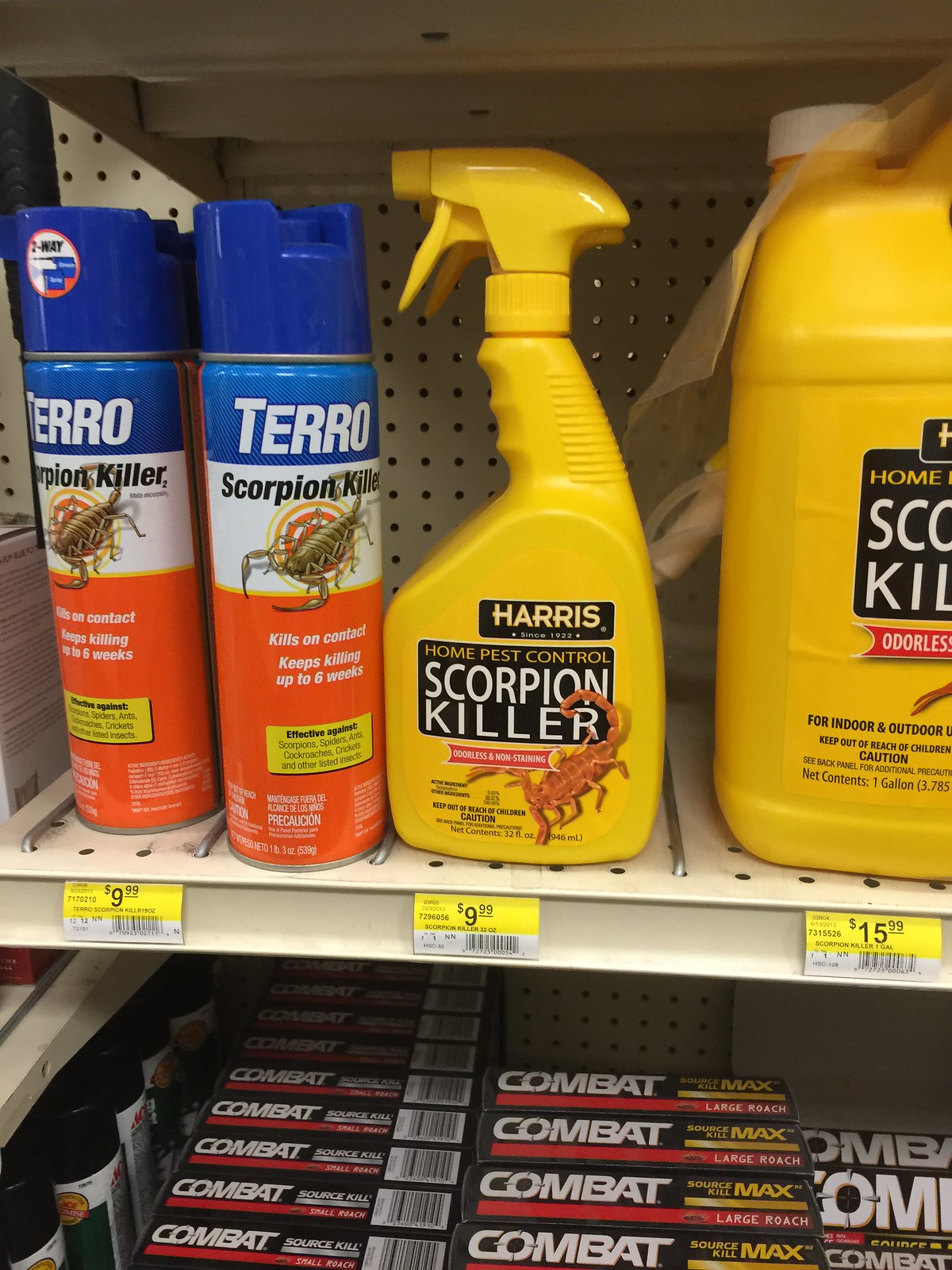The image depicts a store shelf dedicated to Scorpion Killers. Prominently featured on the left are Taro brand Scorpion Killer spray cans, each priced at $9.99. These cans have an eye-catching color scheme transitioning from orange at the bottom, to blue and white in the middle, and finishing in royal blue at the top. Moving right, there is a yellow spray bottle of Harris Home Pest Control Scorpion Killer, also priced at $9.99, notable for its label claiming it is odorless and non-staining, and featuring an image of a scorpion. Further right, there's a larger Harris bottle, similarly yellow-labeled, priced at $15.99. Below these, the bottom shelf displays various packets, including products like Combat Source Kill and Combat Source Kill Max for large roaches, alongside some black-lidded spray cans. The prices are visible on yellow and white tags, and the backdrop is a white perforated display board.